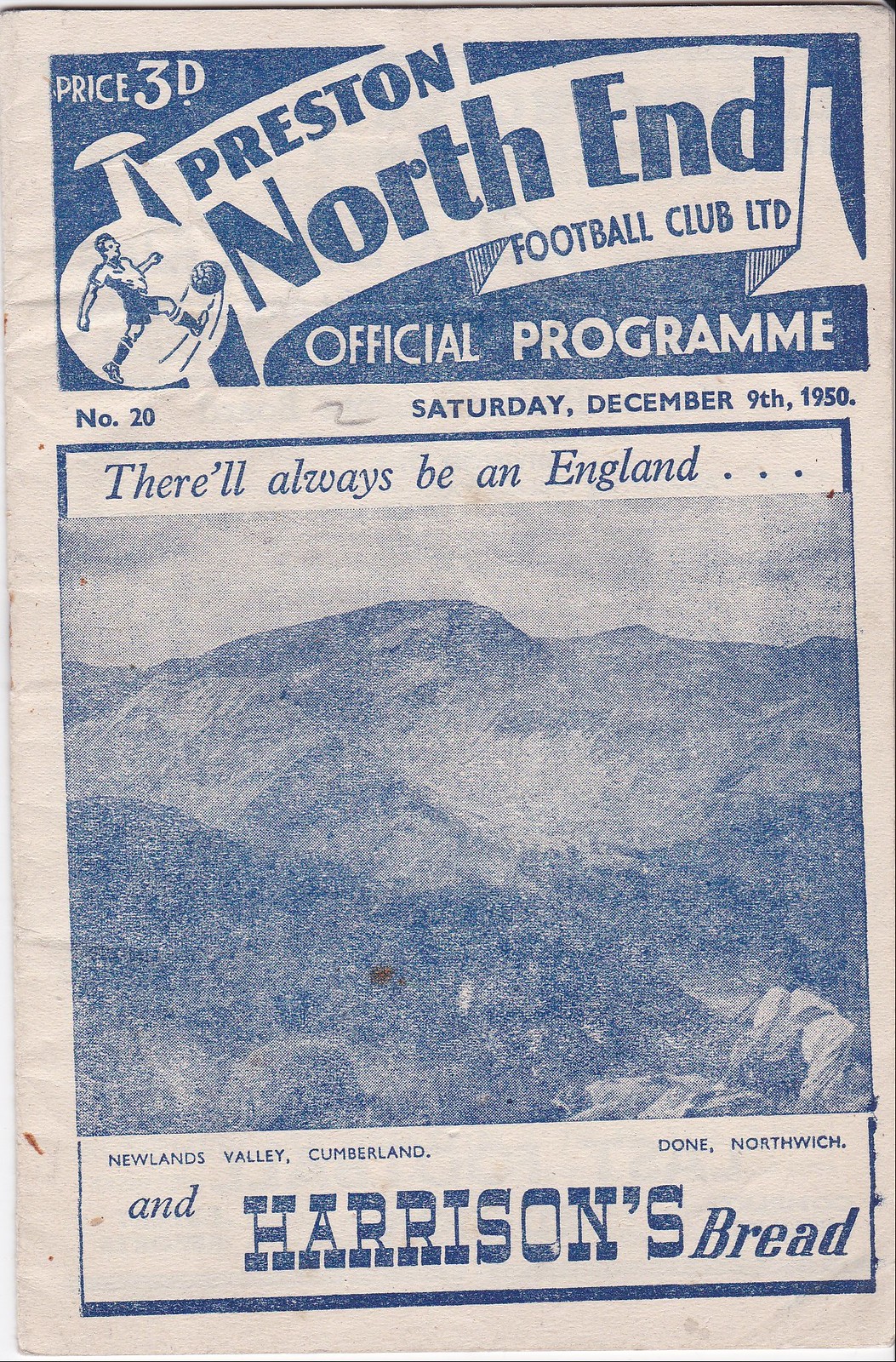This image depicts an aged football program from the Preston North End Football Club, dated December 9th, 1950. The cover, printed on off-white paper, shows signs of water stains, crinkles along the binding, and discoloration. Dominating the top of the cover is a blue banner reading "Price 3D" and "Preston North End Football Club LTD Official Program," adorned with a furled flag illustration and a graphic of a soccer player in mid-kick. Beneath this header, small text indicates that this is issue number 20. The program features a black-and-white, though slightly blue-tinted, photograph of a mountain range, presumably Newlands Valley in Cumberland. Above the photograph, the text "There will always be an England..." is displayed, followed by "and Harrison Bread" in large capital letters below.